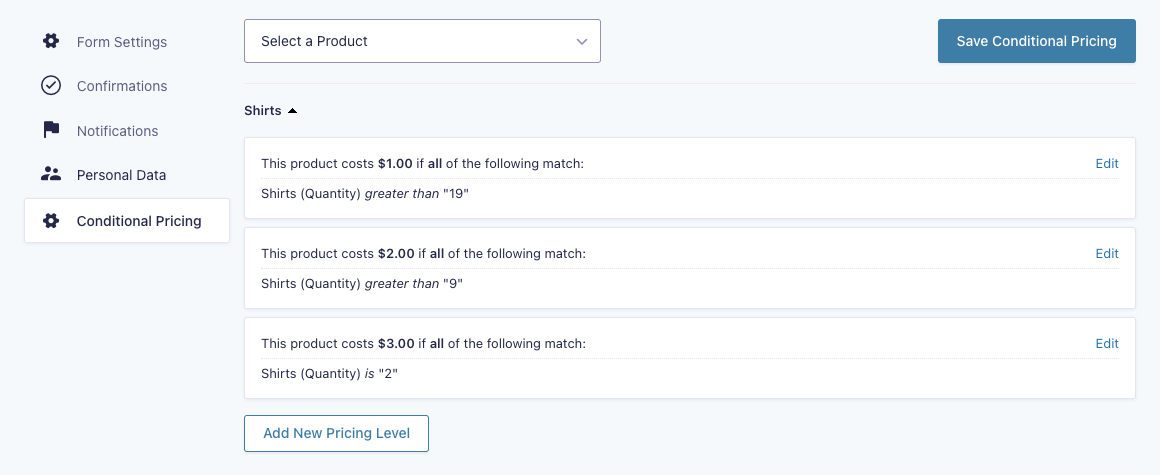Detailed Caption:

This image displays a desktop screenshot of an e-commerce platform's settings page, likely from Shopify or a similar online store interface. The page is focused on setting the price of a product using custom conditional pricing rules. 

**Page Structure and Menus:**
On the left side, a vertical menu is visible with the following options: "Form Settings," "Confirmations," "Notifications," "Personal Data," and "Conditional Pricing." The "Conditional Pricing" option is currently selected.

**Conditional Pricing Section:**
This section contains a dropdown menu labeled "Select a product," which is currently set to "Shirts." Below this, three editable pricing rules are displayed as follows:

1. **Pricing Rule 1:**
   - **Condition:** "Shirts quantity greater than 19"
   - **Price:** "$1"

2. **Pricing Rule 2:**
   - **Condition:** "Shirts quantity greater than 9"
   - **Price:** "$2"
  
3. **Pricing Rule 3:**
   - **Condition:** "Shirts quantity is 2"
   - **Price:** "$3"

Each pricing rule has an "Edit" button to the far right, allowing for modifications.

**Additional Features:**
There is a button labeled "Add new pricing level," which allows the user to create additional pricing conditions. In the top right corner of the page, a "Save Conditional Pricing" button is present for saving any changes made to the pricing rules.

**Design and Layout:**
The background of the page is entirely white, giving it a clean and minimalistic look. The layout is formatted for desktop use, with no visible logos to indicate the exact platform being used.

This detailed setup allows users to tailor product pricing based on specific conditions, offering flexible options for managing sales and inventory.